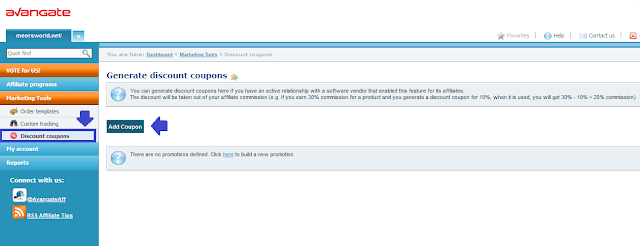The image depicts the interface of a website named "Evengate," with the site's logo prominently displayed in red text at the top left corner. Directly beneath the logo is a search bar for easy navigation. Below the search bar, there is a vertical menu listing several options, including "Vote for USI," "Affiliate Programs," "Marketing Tools," "Order Templates," "Custom Trading," and "Discount Coupons," the latter of which is currently selected.

Upon selecting "Discount Coupons," the main section of the interface displays a title "Generate Discount Coupons" alongside an "Add" button. At this point, no coupons appear to have been generated or added. These coupons would typically be used to avail discounts on various offerings available on the site.

The menu on the left also includes additional options like "My Accounts," "Report," and "Connect with Us," each of which provides various tools and functionalities to enhance user interaction and management. 

On the top right corner of the interface, there is a "Favorites" menu, allowing users to bookmark their preferred sections or features for quick access. Next to it are menus for "Help" and "Contact Us," providing assistance and customer support options. The interface is completed with a "Logout" button, facilitating a secure exit from the user account.